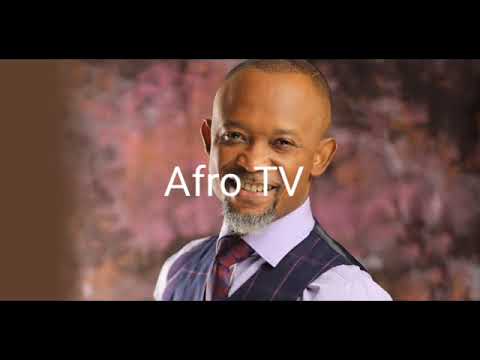The image features a headshot of a middle-aged black man with brown skin and a goatee, against a blurred, multicolored background dominated by hues of pink, brown, and tan. The background is darker in the upper right corner and includes a trim of brown along the left edge. The man, centrally positioned and looking directly at the camera with mostly closed eyes and a slight squint, has very short hair. 

He is dressed in a sophisticated ensemble comprising a light purple, collared shirt that reaches up to his chin, a blue vest adorned with purple stripes, and a purple and black tie. Superimposed across his face, the text "AFROTV" is prominently displayed. The image is cropped just below his shoulders, creating a focused composition. Aesthetic black lines create borders above and below the image, enhancing the visual structure. The overall impression suggests the image is part of an advertisement, possibly for a TV show or network.